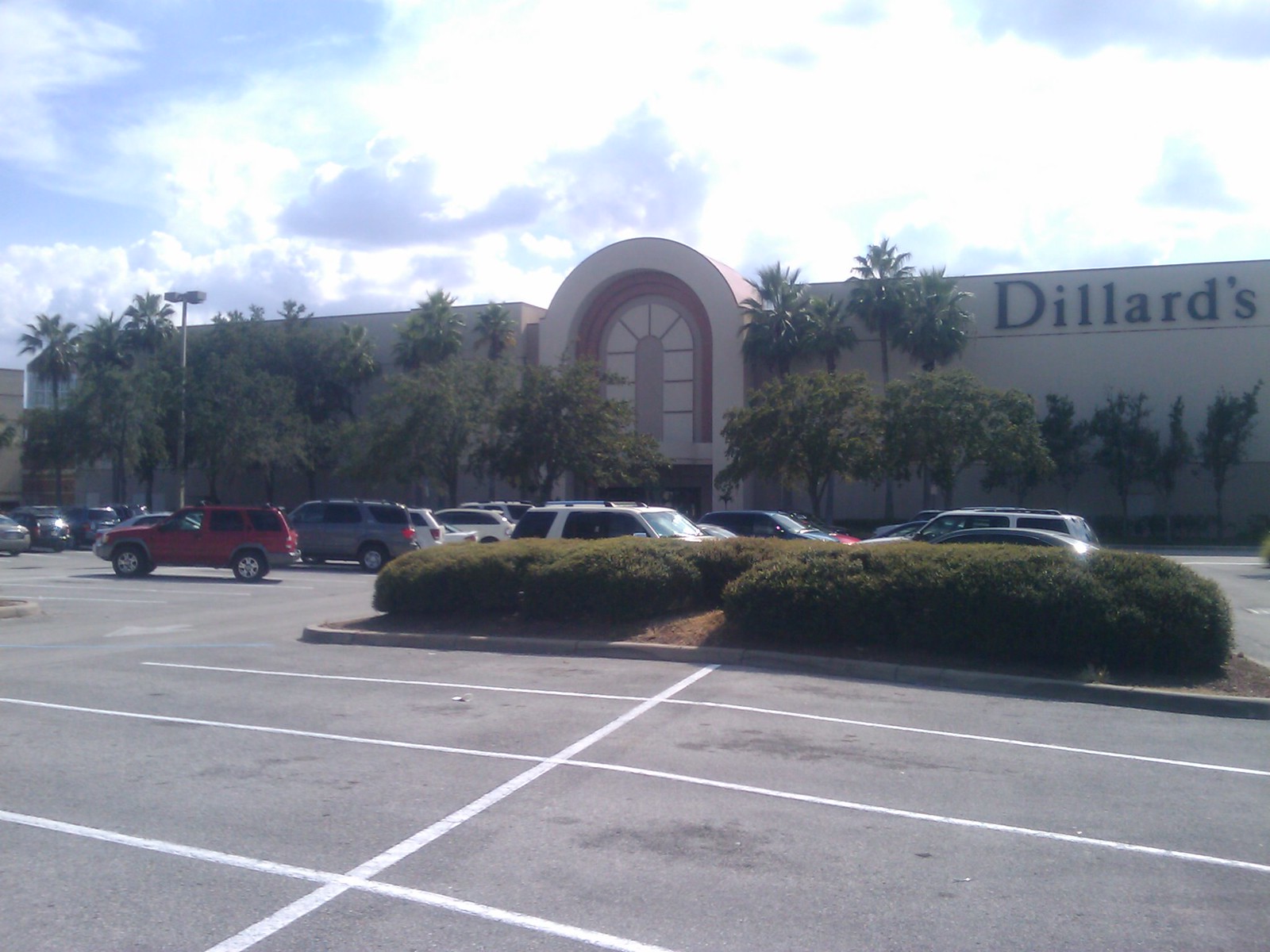This photograph captures the front façade of a Dillard's department store, set against a bright daytime sky adorned with fluffy white and occasional gray clouds. The store is housed in a long, light beige, stone-like building. Prominently displayed in the upper right corner of the building, "Dillard's" is written in bold black letters. Central to the image is a grand archway above the store's entrance, constructed of white stone with red accents and featuring a star-like pattern. 

Flanking the building are numerous palm trees, with shorter, younger trees interspersed among them. In the foreground stretches a vast asphalt parking lot, neatly marked with white parking lines. Several vehicles are parked closer to the store, likely belonging to customers or employees. A rectangular island with wood chips and low-lying bushes punctuates the parking lot. Additionally, a street lamp and some surrounding buildings are faintly visible in the background, completing the scene of this bustling retail environment.